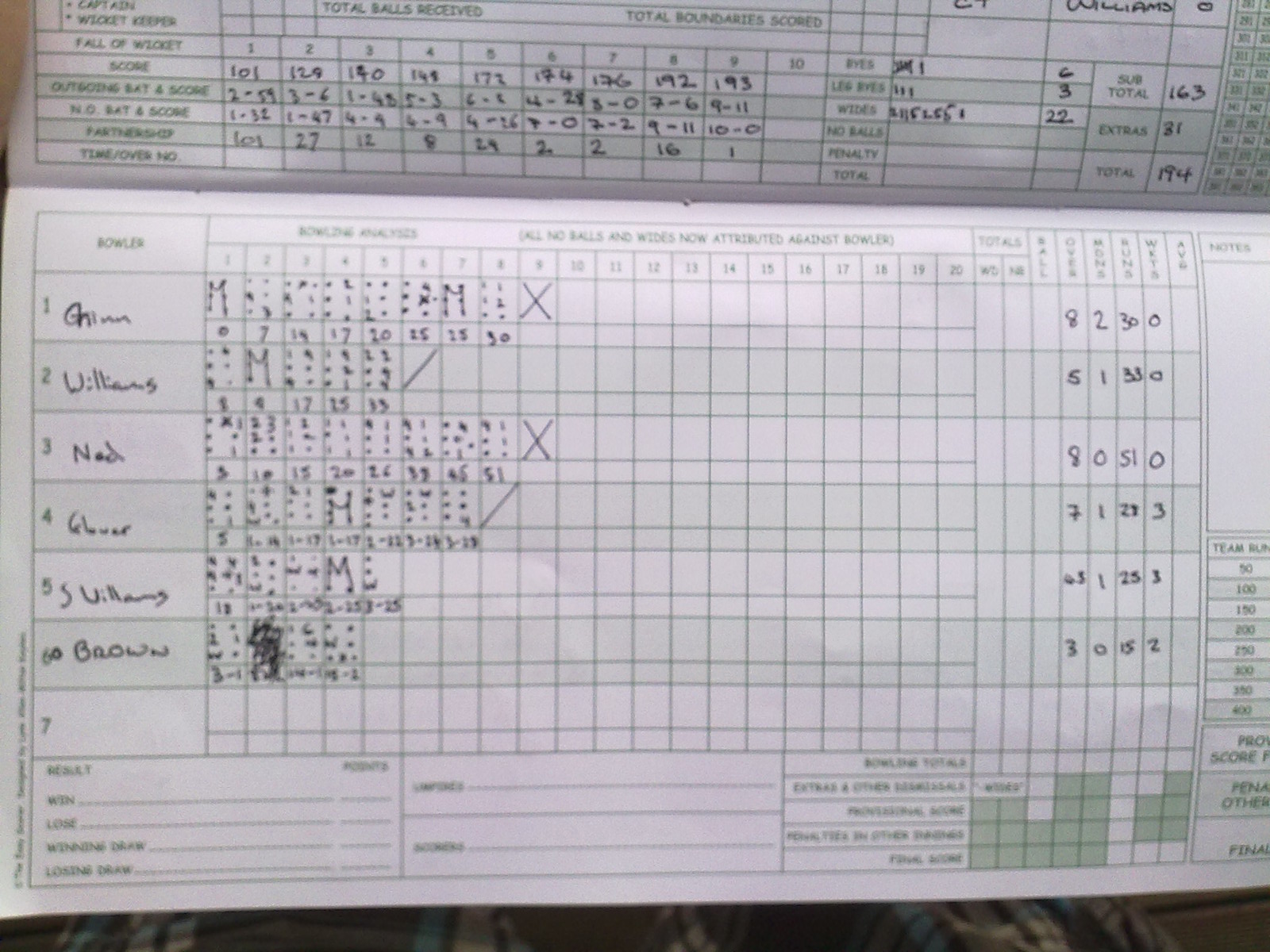The image is a horizontal, rectangular photograph of a white piece of paper that resembles a black and white photo but includes green columns and grids. This paper appears to document bowling scores. Six bowlers' names—Gian, Williams, Ned, Glover, S. Williams, and Brown—are listed along the left-hand side, numbered from one to six. Each bowler's scores are recorded in the corresponding columns to the right, written in very small, black pen text, making the details difficult to read. The image only shows the lower half of the bowling score sheet, as the upper part is mostly cut off. The green columns and grids structure the sheet, with additional black writing populating the boxes.